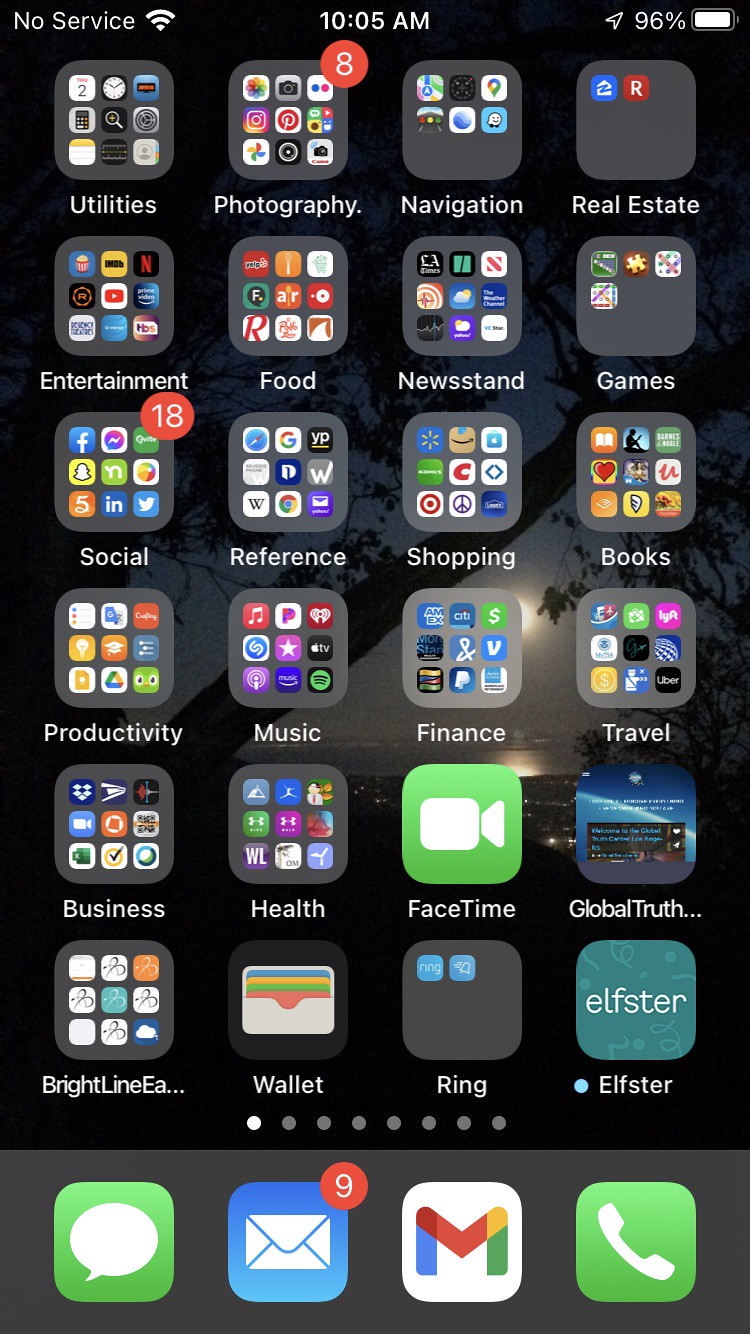This is a detailed screenshot of an iPhone home screen. At the top, the status bar indicates no service with Wi-Fi connected, the time displayed is 10:05 AM, and the battery level is at 96%. The dock at the bottom features the Messages app, Mail app with 9 notifications, Gmail app, and the Phone app. The wallpaper showcases a serene night scene of the moon shining over what appears to be an ocean, viewed through the silhouette of a large tree, with some lights from a building visible below.

The home screen is organized into six rows, each containing four folders or apps as follows:

1. **Top Row:**
   - Utilities
   - Photography
   - Navigation
   - Real Estate

2. **Second Row:**
   - Entertainment
   - Food
   - Newsstand
   - Games

3. **Third Row:**
   - Social
   - Reference
   - Shopping
   - Books

4. **Fourth Row:**
   - Productivity
   - Music
   - Finance
   - Travel

5. **Fifth Row:**
   - Business
   - Health
   - FaceTime
   - Global Truth

6. **Bottom Row above the Dock:**
   - Brightline Eats
   - Wallet
   - Ring folder
   - Elfster

The presence of dots at the bottom suggests there are additional pages of apps available.